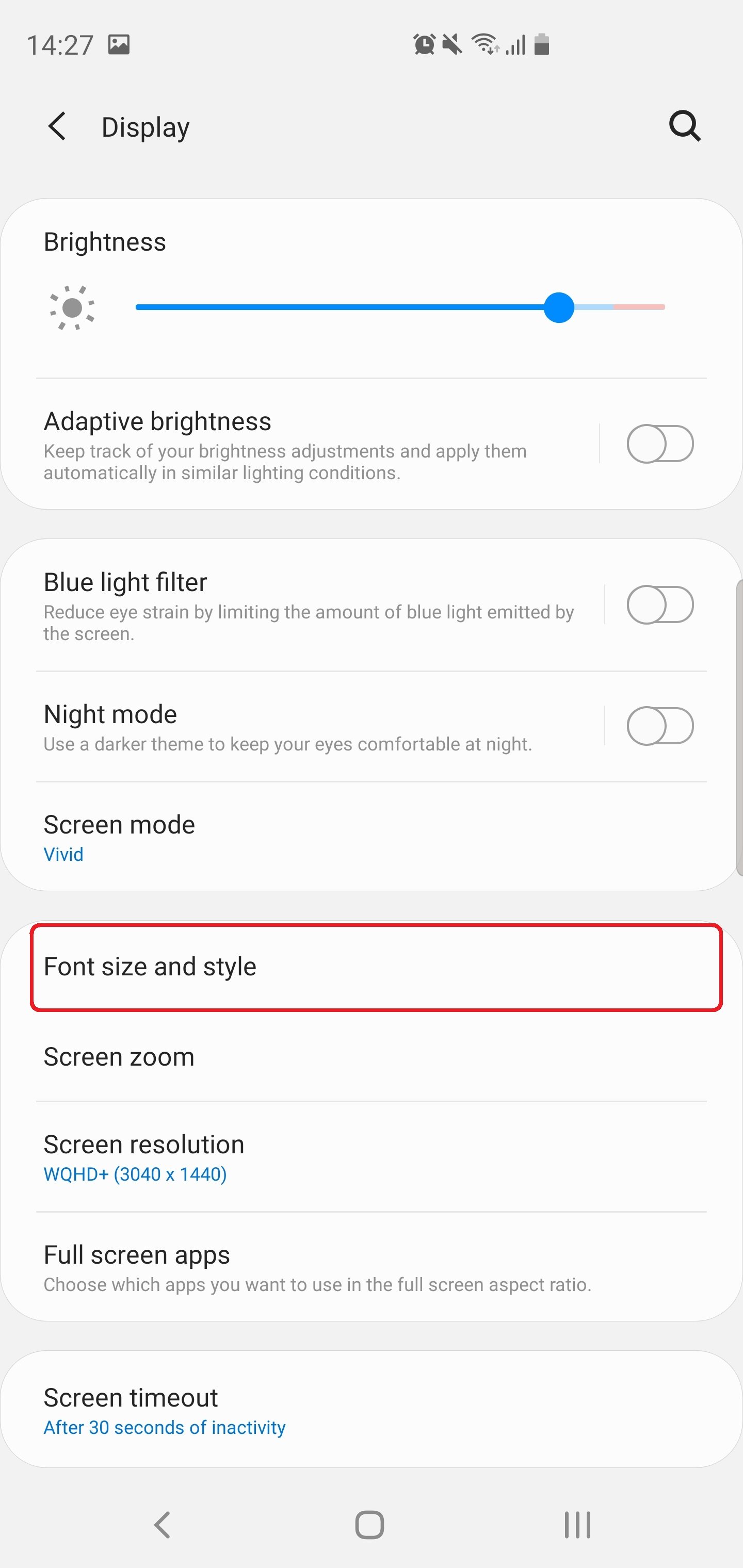A detailed screenshot from a smartphone's settings menu, showcasing the 'Display' tab in light mode. At the top of the screen, it displays the time as 14:27, with the alarm clock active, but the sound is off. The phone has a full Wi-Fi connection, strong network signal, and a battery level at approximately 66%. The header section includes a back arrow, the title 'Display,' and a search function. 

Just below that, the brightness adjustment bar is visible, set to about 70-75% of its maximum level. The 'Adaptive brightness' setting, which automatically adjusts brightness based on lighting conditions, is turned off. The 'Blue light filter' setting, aimed at reducing eye strain by limiting blue light, is also turned off. 'Night mode,' designed to provide a darker theme for comfort at night, is similarly deactivated.

The 'Screen mode' is set to 'Vivid.' The option 'Font size and style' is highlighted with a red box, drawing attention to it. Further down are options for 'Screen zoom,' 'Screen resolution,' 'Full screen apps,' and 'Screen timeout.' No other significant details are noted in this comprehensive capture of the phone's display settings.